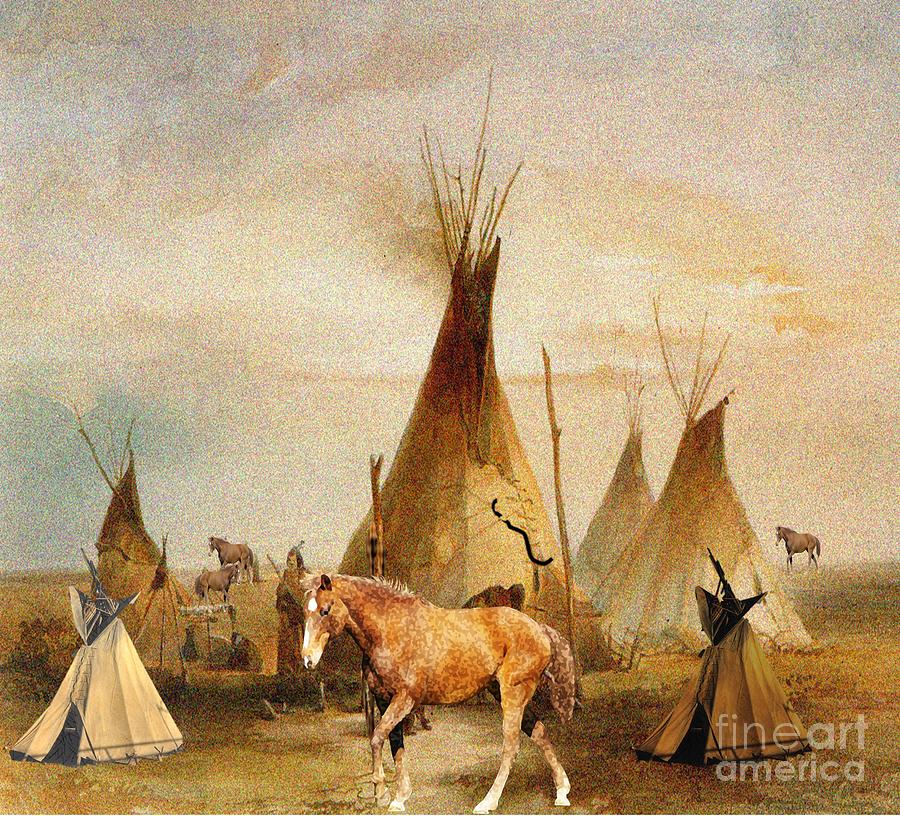This evocative painting by Fine Art America captures a serene scene of a Native American village, likely rendered in watercolor with a grainy texture that adds depth and an aged feel. The setting features six traditional Native American dwellings, or tipis, with the largest positioned prominently in the center. This central tipi exudes a sense of community, with its structure of poles extending upwards and tied to form its characteristic conical shape. 

In the foreground, a reddish-brown horse stands majestically, its white-marked face and legs contrasting against its dark mane and tail. Surrounding the central tipi are two small tipis in the foreground and three other medium-sized tipis further back. Each tipi displays a unique arrangement of poles at the top, some with a hint of smoke suggesting fires burning within.

The backdrop is an expanse of dry, brownish grasslands beneath a striking sky that transitions from shades of blue to mottled white and gold, creating a dramatic atmosphere. Scattered throughout the scene are additional horses, including three brown ones in the far background, and a singular figure who appears to be watching over the village, possibly a Native American adorned with traditional attire.

The overall palette of the painting leans towards muted sepia tones, enhancing its nostalgic and historic ambiance. At the bottom right corner, the transparent white logo of Fine Art America subtly asserts its brand without detracting from the visual storytelling.